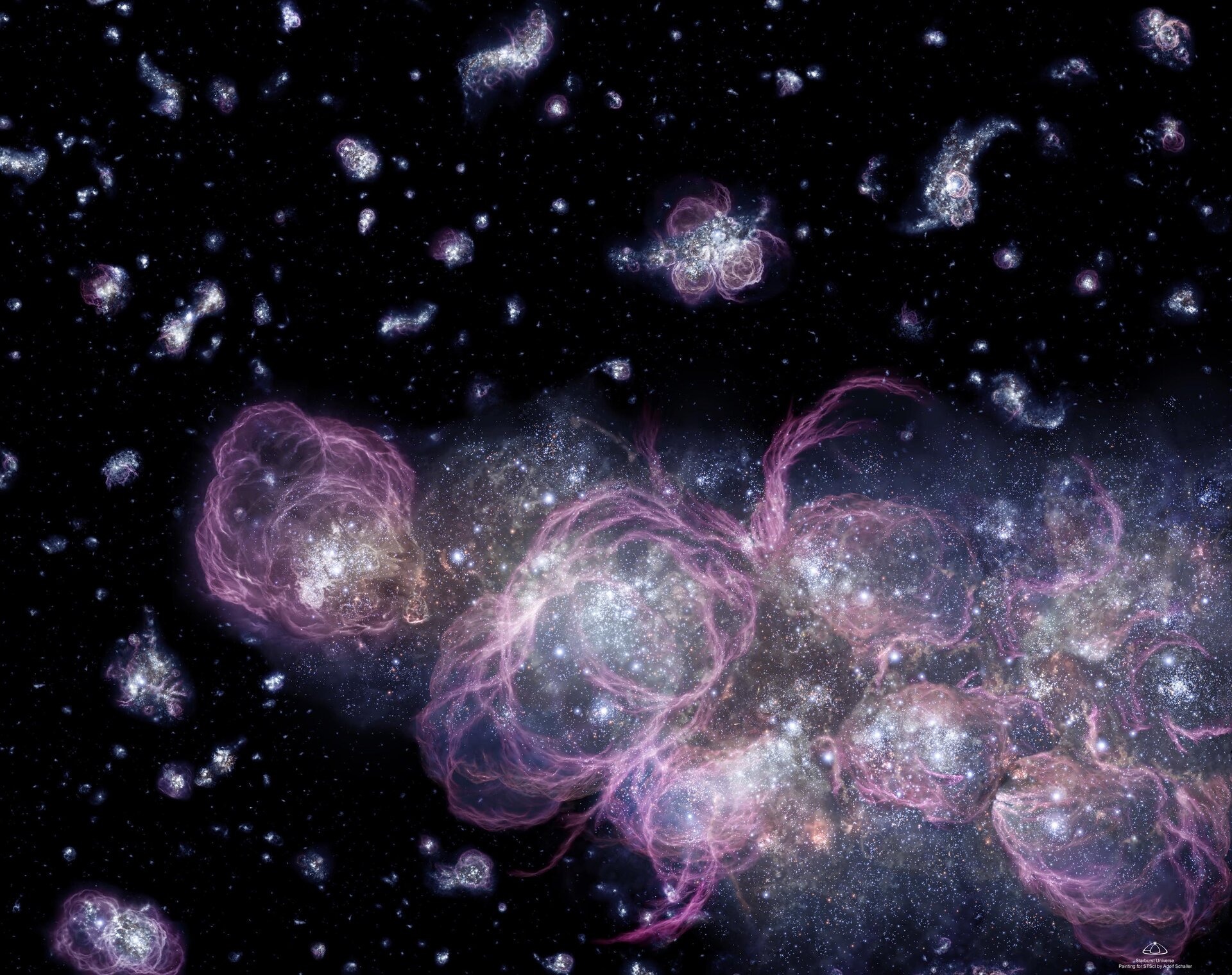The image is a detailed, computer-generated depiction of a celestial scene, resembling the deep ocean or outer space. It features what could be interpreted as galaxies or translucent deep-sea creatures, floating against a super dark background that suggests either the ocean depths or the expanse of space. Centrally, the image has a cluster of large, swirl-like purple creatures or nebulae, densely packed, with tendrils and striations extending from the right to the left. These central figures are bigger and more prominent, creating a striking focal point. Scattered across the rest of the image are smaller, similar forms that diminish in size with distance, evoking a sense of depth and vastness. The background is predominantly black, dotted with thousands of tiny, bright stars or light points, further enhancing the illusion of a star-filled sky or phosphorescent underwater life forms. A small, unreadable logo is placed somewhere on the image. The scene is an intricate blend of natural and cosmic elements, creating a mesmerizing and otherworldly visual experience.